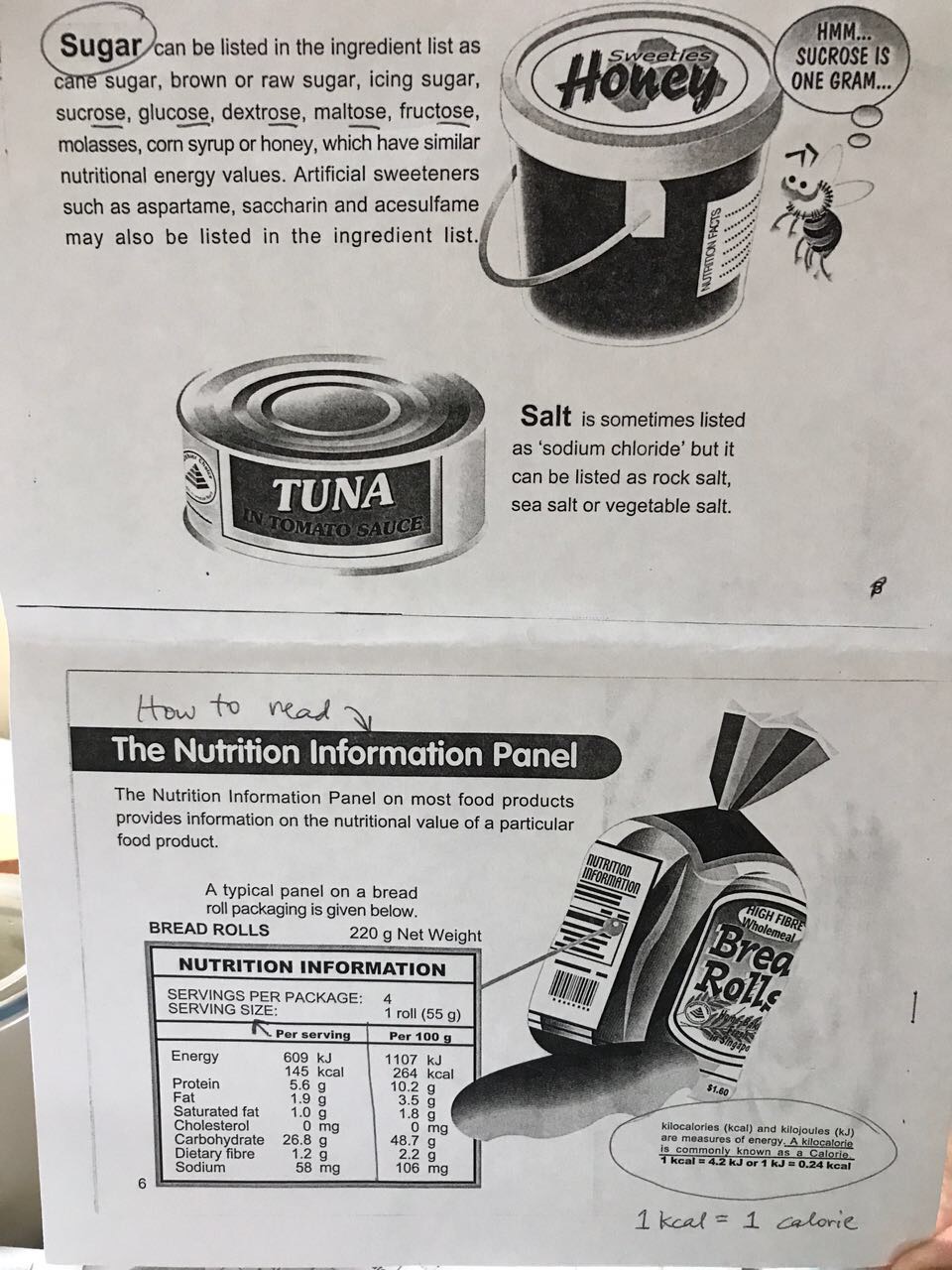The image is an informative illustration about nutrition, focusing primarily on educating the viewer about different names for sugar and how to read nutritional labels. At the top, it explains that sugar can be listed under various names, including cane sugar, brown or raw sugar, icing sugar, sucrose, glucose, dextrose, maltose, fructose, molasses, corn syrup, and honey. Accompanying this text is an image of a honey jar with a bee next to it, indicating that sucrose is one gram. Below this, there's an illustration of a tuna can labeled with details about salts, such as sodium chloride. Further down, the image provides a comprehensive guide on how to read a nutritional information panel. This section features a packet of bread rolls with an informative arrow pointing to its nutritional label, explaining each component. An additional note clarifies that one calorie equals one kilocalorie. The entire illustration is rendered in black and white, enhancing the educational focus of the content.